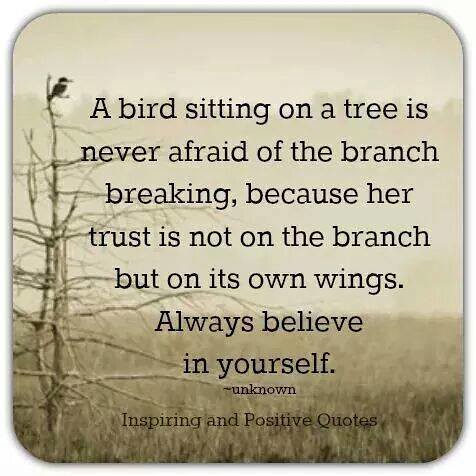This square image, with softly rounded corners and a subtle gray shadow surrounding it, features a light brown-toned photograph. The bottom of the image depicts a blurry, grassy area, while a thin, leafless tree stands on the left side, reaching long barren branches towards a misty, white-and-brown sky. At the top of the tree perches a small black bird. Overlaying the right side of the photo in black text is an inspirational quote: "A bird sitting on a tree is never afraid of the branch breaking because her trust is not on the branch, but on its own wings. Always believe in yourself." This quote is attributed to unknown and is presented by "Inspiring and Positive Quotes."